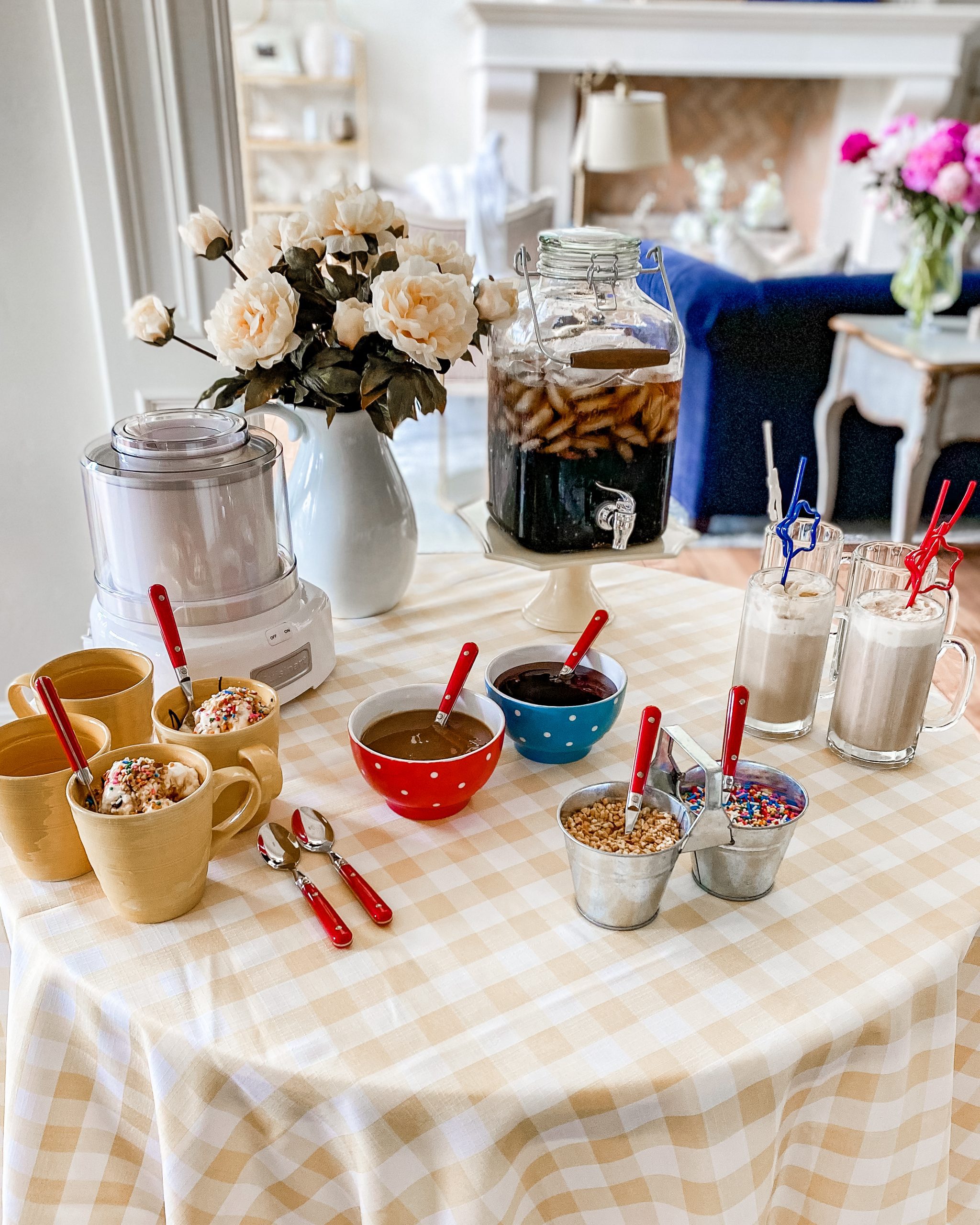The image depicts a small round table adorned with a honey and white checkered tablecloth, set in what appears to be an elegant room. The table features a charming assortment of items, evoking a delightful ice cream station. There are four tan mugs on the left side, two of which are filled with ice cream topped with sprinkles. Additionally, there are four mugs on the right, containing what looks like root beer floats with decorative twisty straws—one blue, one white, and two red. Two silver metal pails hold assorted sprinkles, one with multicolored sprinkles and nuts. The table also hosts two ceramic bowls: a red bowl with white dots and a blue bowl with white dots, both appearing to contain sauces, likely chocolate.

In the center lies a white vase brimming with white roses, lending a touch of elegance. To its left, there is a sturdy, glass beverage dispenser on a white, octagonal stand, filled with a dark liquid, possibly cola, root beer, or apple cider with floating fruit slices. The table also contains various matching spoons with bright red handles, scattered on the table and within the mugs and pails.

Background details include a neatly arranged living room. A blue couch sits near the table, beside a white ornate end table holding a vase of pink, red, and white flowers. There is a gold or brass lamp, a light brown shelf with white items, and a large white fireplace featuring a diagonal brick pattern, subtly framing the elegant setting.